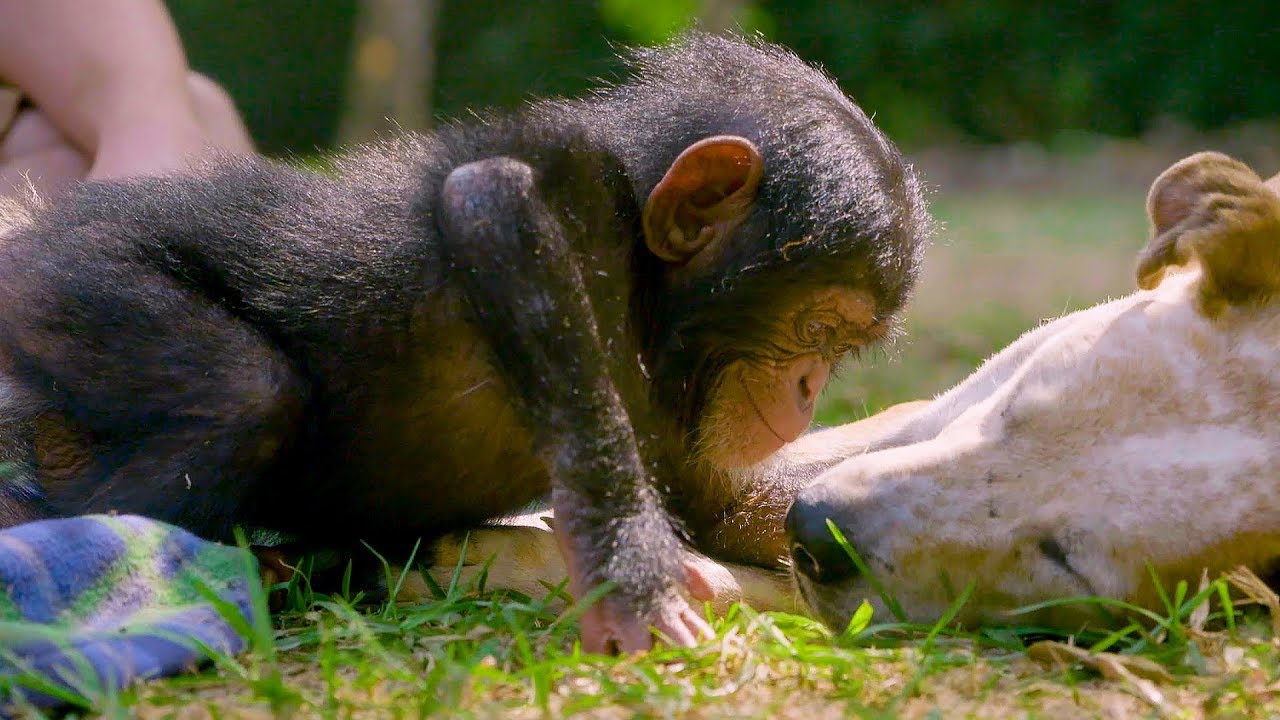In this charming outdoor photograph, a heartwarming scene unfolds with a baby chimpanzee and a large white dog with brown patches and a floppy ear. The dog, lying in the grass with its eyes closed and head resting wearily on the ground, seems at peace under the midday sun. In front of the dog, the young chimpanzee, appearing to smile, leans in close as if about to plant a gentle kiss on the dog's nose, showcasing a tender moment of interspecies affection. To the right of the little chimp, a piece of a plaid blanket with blue, white, and green patterns is visible on the grass. In the background, we can see a person whose crossed leg and part of their arm peek into the frame, suggesting they are observing the affectionate interaction from a distance. Blades of grass in the immediate foreground add depth to this sweet and serene image.